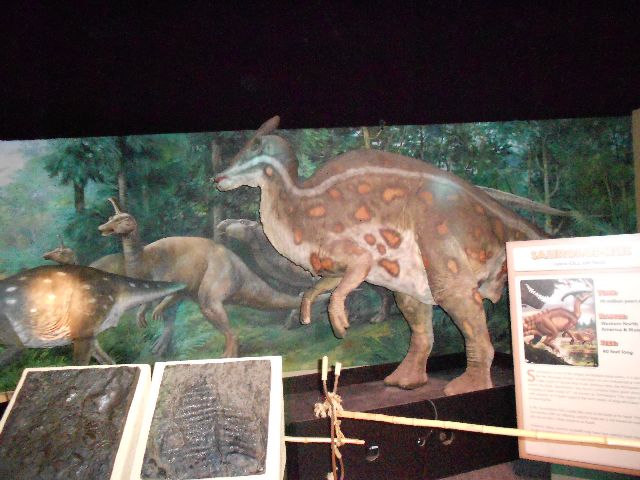The image depicts an indoor exhibit, likely within a museum or a zoo, centered around a dinosaur-like statue. The central figure resembles a hybrid creature with kangaroo-like posture, featuring a brown body with a beige underside, orange-brown spots, and distinct anatomical features like small front limbs and larger hind legs. Its head, reminiscent of a deer, is marked by a white stripe running from the nose to the tail.

In the background, various other animal representations and tree-like elements create a forest-like scene. Two white, unreadable signs are visible at the bottom left of the image, while the bottom right corner features a similarly unreadable informational sign about the dinosaur statue. A rope barrier stretches across the middle of the scene, indicating restricted access. The upper portion of the image shows a black band, contributing to the indoor ambiance of the exhibit.